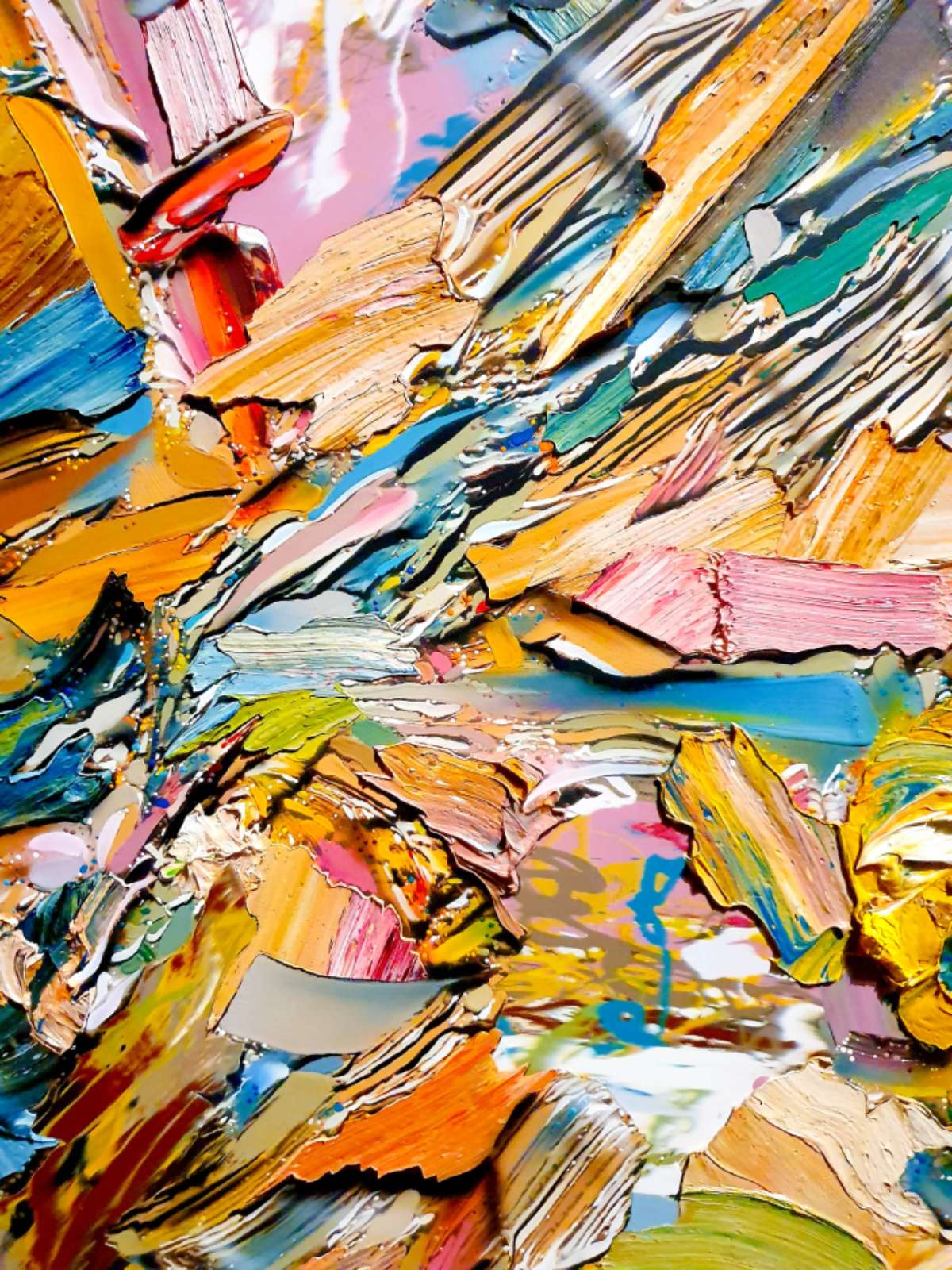The image is an abstract, vividly colorful painting characterized by thick, layered brush strokes. The composition features a multitude of colors, including red, pink, yellow, blue, green, black, brown, lime green, dark blue, bright red, white, aqua blue, and shades of orange and tan. The paint appears to be applied in a highly textured style, creating a multidimensional effect with areas that look cracked and chipped, revealing the layers beneath. In the middle of the image, there is a noticeable horizontal blue line. Near the top left, there's a prominent, irregular shape in shades of orange-red, and the top right contains a smaller patch of gray. The entire canvas is filled with chaotic, random shapes and strokes, giving it a dynamic, energetic feel. There is no identifying information such as an artist's name, location, or date visible in the painting, and no figures or discernible objects are present. The painting may be a physical artwork or a digital creation emulating traditional painting techniques.